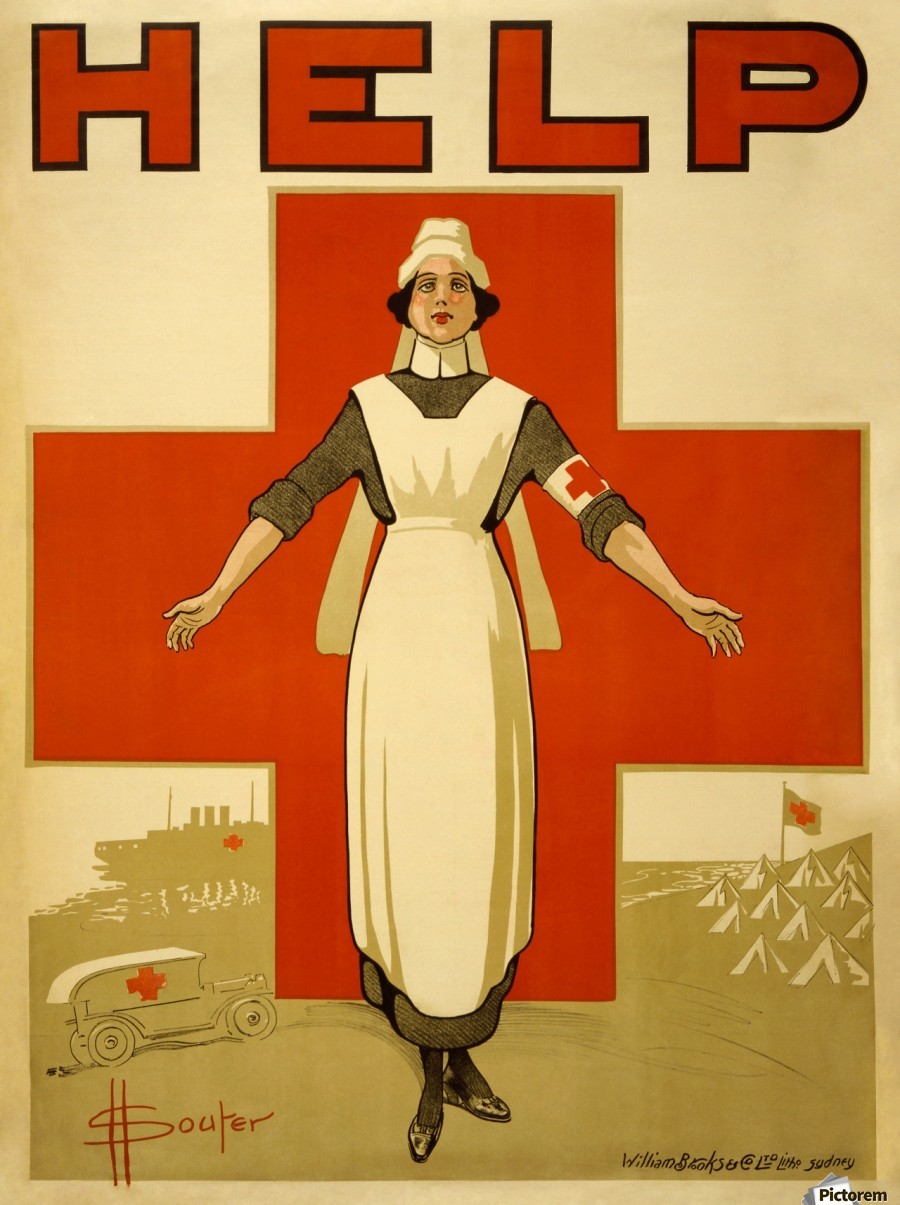The image is an illustration of a vintage wartime poster prominently featuring a nurse set against a striking red cross background. The nurse, standing at the center with arms outstretched, is dressed in a traditional black shirt topped with a long white frock that extends into a gown, accentuated by black trim at the bottom of the skirt. She wears a white headgear and black shoes, with a distinct white patch on her left arm bearing a red cross. Her facial expression conveys a somewhat dazed or earnest emotion. At the very top of the image, the word "HELP" is boldly displayed in red block letters. The lower portion of the image depicts a detailed military scene, including a brown military tank, a Red Cross jeep in motion, a ship, several tents, and a flag with the red cross symbol. The signature "SOUTER" appears in the bottom left corner, while additional black text can be found at the bottom right, reinforcing the theme of Red Cross or medical assistance during wartime.